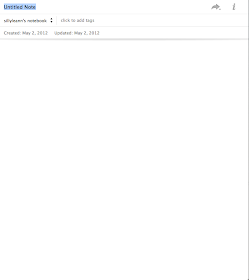The image depicts a blurry website interface that is difficult to read. Central to the image is a blue box containing black text that appears to say "Untitled Note." Adjacent to this box, on the same row to the right, is a thin gray vertical line separating it from a gray right-pointing arrow. This arrow leads to a blurred vertical gray area. Following this, there is text including an apostrophe 'S' and a colon, with the instruction "Click to add tags" displayed in gray text.

Below this section, the website shows a row with the text "Created May 2nd, 2012" and another similarly blurred date that seems to be "May 2nd, 2012," separated by another thin gray horizontal line. A vertical gray line runs along the right side of this section, and the rest of the image remains blank.

This detailed structure suggests an interface for note-taking or task management, although the blurriness obscures specific functionalities or context.